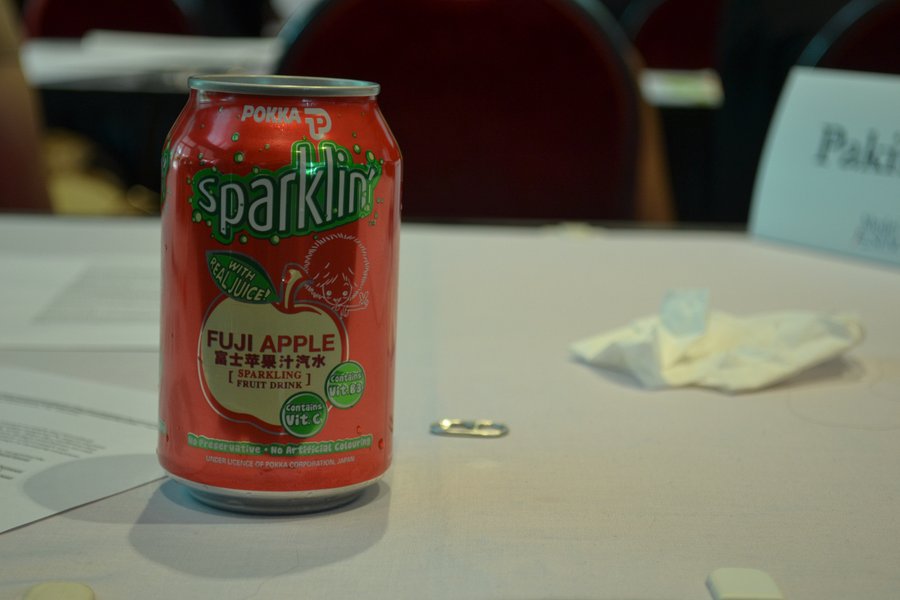In the image, a single can sits prominently on a light gray table, accompanied by a few other objects. The can is positioned in the center and is a vibrant red, branded with "POKKA" in gray lettering. The top of the can is silver. The label features a sparkling white text set against a green background, stating “with real juice.” Depicted on the can is the design of a white apple encased in a red outline, with the words "Fiji Apple" displayed in red. Additional text on the can includes information in a non-English language, along with the phrases "Sparkling Fruit Drink," “Contains Vitamin C,” and another unspecified vitamin, both highlighted in green circles, with more green text below that.

To the left of the can lies a tan-colored object and two white pieces of paper. To the right, there is a white tissue and the cap of the soda situated in front of the can. The table is light gray, providing a neutral backdrop to the objects. In the far background, the back of a dark brown and black chair is visible on the right side. The left side of the image fades into blurriness, adding to the focus on the can and surrounding objects. At the very bottom right of the image, a small gray square is noticeable, adding a subtle detail to the composition.